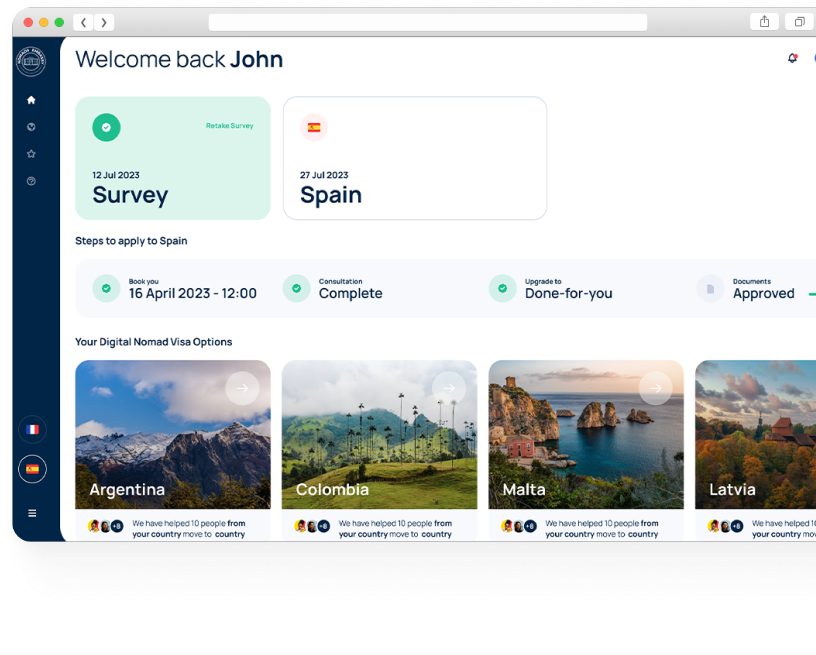The top left corner features the typical window control buttons in red, yellow, and green, which correspond to close, minimize, and maximize functions respectively. Below, there are navigation buttons for back and forward, followed by a search bar. Additionally, there are two more buttons: one with a square and an upward arrow, and another with multiple layered squares.

A blue sidebar displays two flags: one with vertical blue, white, and red stripes (likely the flag of France), and another with horizontal red, yellow, and red stripes (likely the flag of Spain). The sidebar also greets the user with "Welcome back, John," and lists various surveys and statuses: 

- "Survey 12 July 2023" with a check mark
- "Spain 27 July 2023"
- "Steps to apply to Spain 16 April 2023 - 12"
- "Complete"
- "Done for you"
- "Approved."

At the bottom, there are images presumably showcasing different destinations, labeled under "Your Digital Nomad Visa Options," with country names like Argentina, Colombia, Malta, and Latvia.